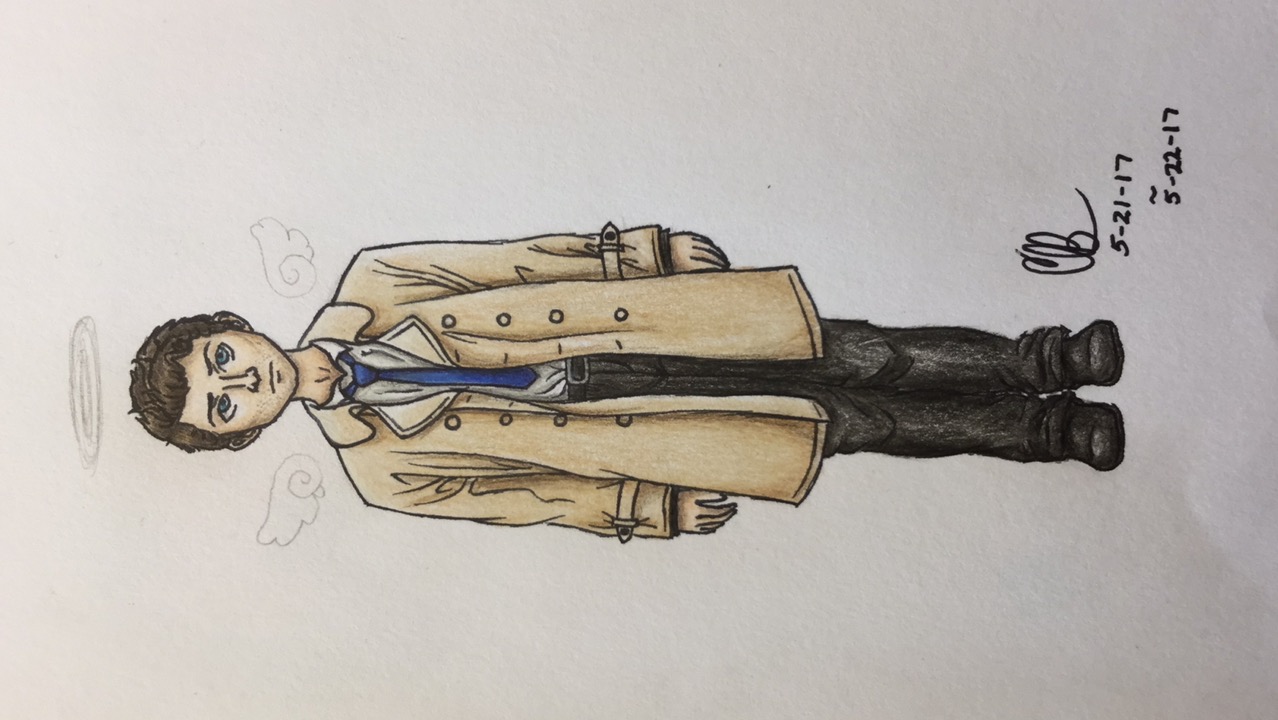This is a meticulously detailed colored drawing of a young boy, likely around 14 years old, set against a white background. The boy stands front-facing with his legs together, his straight arms down at his sides, hands visible from beneath a loose, light beige overcoat that hangs over his shoulders and extends just above his knees. This trench coat features four buttons on either side of the wide-lapeled breast, and bands around the cuffs. Underneath, he wears a white collared shirt with a blue tie, visible belt, dark pants (possibly blue jeans), and dark shoes. The boy has a Caucasian complexion, thick brown hair with ears peeking out, blue eyes looking to his left (our right), and a neutral, slightly sad expression. Above his head is a lightly sketched halo, and similarly sketched wings float behind his shoulders, suggesting an angelic motif. The drawing is signed with initials, likely "CB," and dates "5-21-17" and "5-22-17" near the lower right area beside his left foot. The overall style is more serious than cartoonish, with a blend of realism and artistic interpretation.